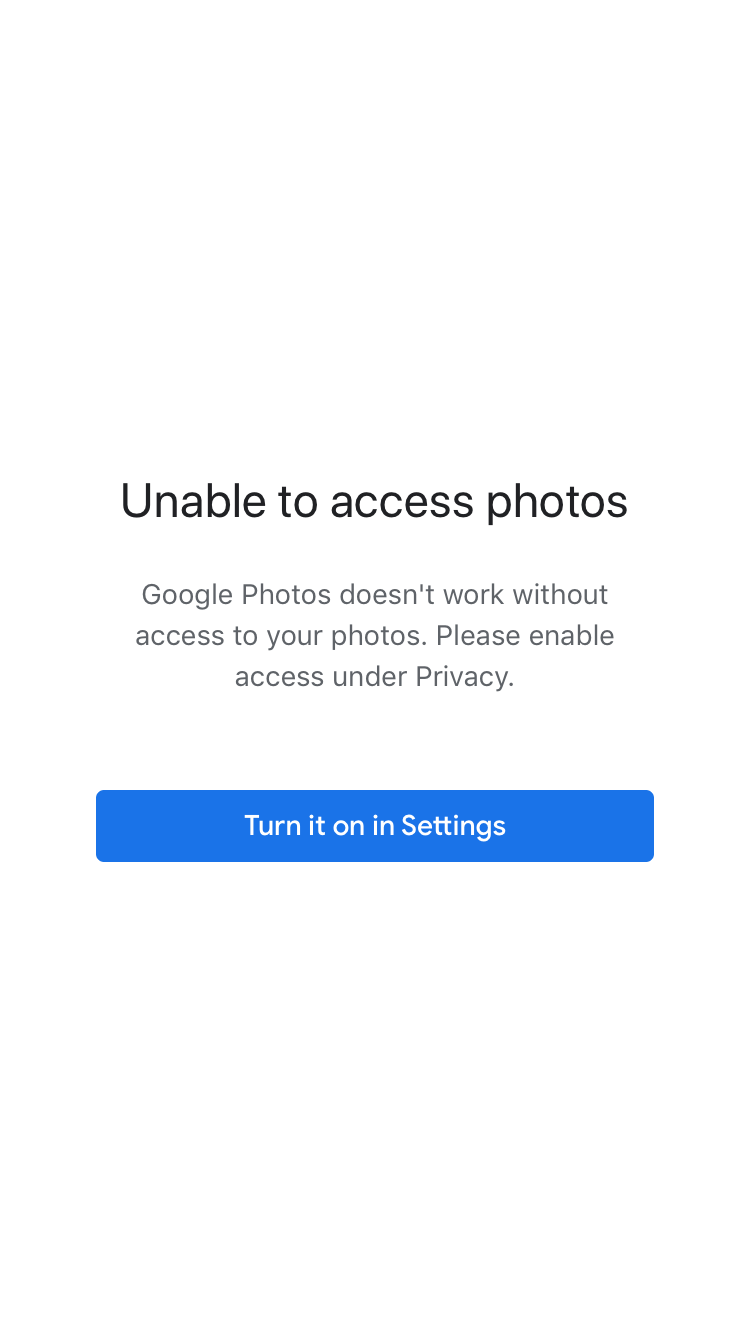This is a screenshot from a slim mobile device, capturing a notification from Google Photos. In the center of the white background, the prominent text in bold, black letters reads "Unable to access photos." Directly below, in smaller, gray letters, it states "Google Photos doesn't work without access to your photos. Please enable access under privacy." Beneath this message, a blue button says "Turn it on in settings." All text and elements are centrally aligned within the white rectangle, creating a clean and focused layout. The background's bright white color contrasts sharply with the text and buttons, highlighting the notification's urgency and clarity.